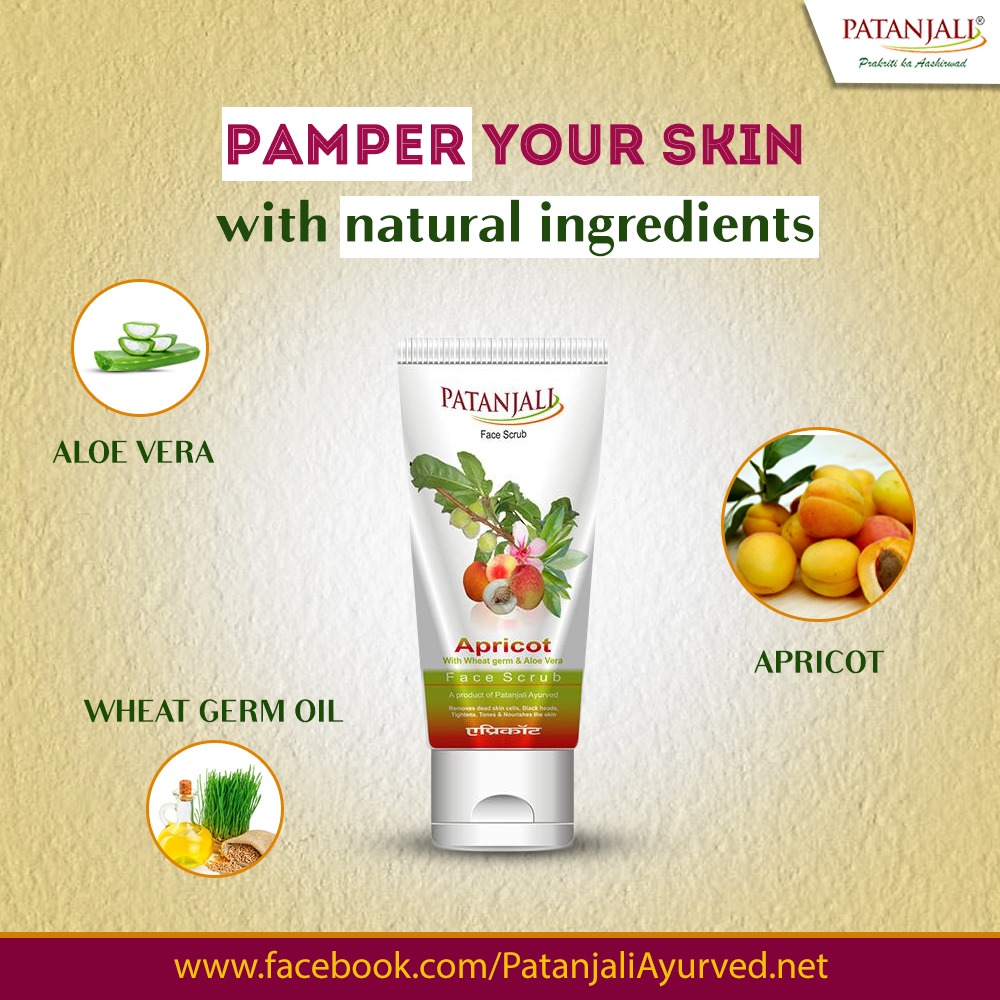This vibrant advertisement for Patanjali's apricot face scrub vividly promotes the product's natural ingredients with the tagline "Pamper your skin with natural ingredients." The focal point of the ad is a centrally-placed squeeze tube of the face scrub, adorned with green and red hues. Surrounding the tube are images of the key ingredients: a cut aloe vera leaf, a visual of wheat germ seeds and oil, and a cross-section of an apricot. Each ingredient is displayed in its respective circle, highlighting the face scrub’s composition of aloe vera, wheat germ oil, and apricots. At the bottom of the ad, a Facebook handle is provided for viewers to obtain more information or make a purchase, offering both convenience and connectivity.